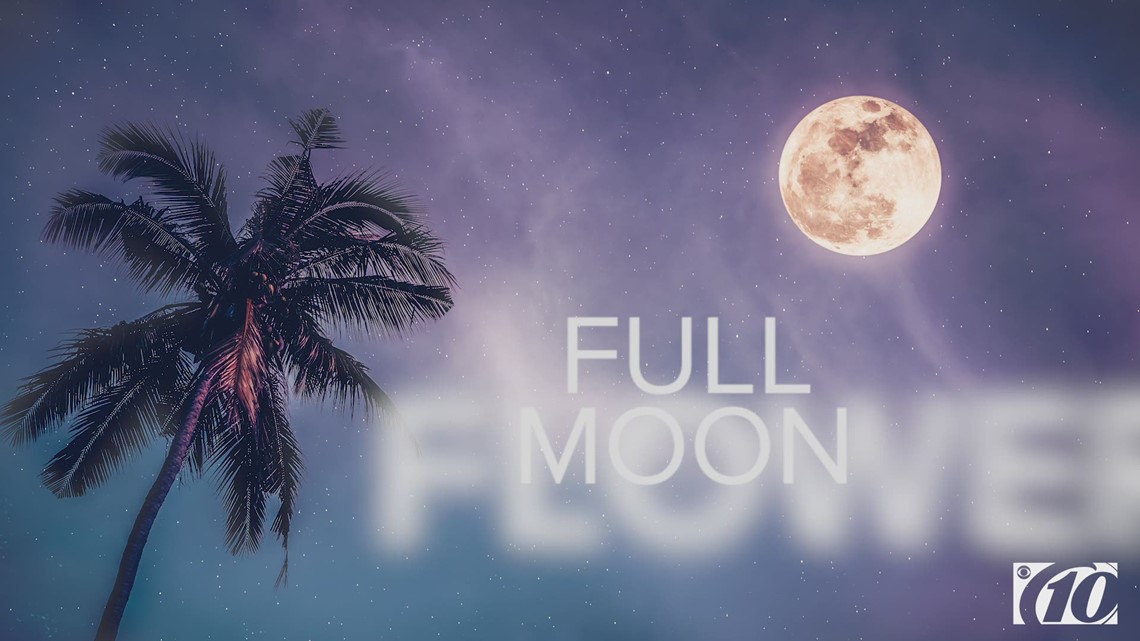In the image, we see a captivating night sky dominated by a full moon positioned in the upper right corner. The foreground features a palm tree extending from the bottom left, with its trunk and leaves stretching towards the middle of the frame. The sky is a rich mix of deep blue, purple, and black hues, sprinkled with stars. The scene has an ethereal quality, possibly digitally enhanced or a screen capture from a TV show or advertisement.

The text "FULL MOON" is prominently placed slightly off-center towards the right. Below and somewhat behind it, the word "FLOWER" is faintly visible in cloud-like skywriting, with parts extending beyond the image’s right edge. Near the bottom right corner, a small box contains the number "10" with an accompanying symbol, adding to the enigmatic ambiance of the image.

The color palette includes shades of blue, purple, black, white, green, brown, and tan, contributing to the night-time atmosphere. Overall, this image seamlessly blends natural elements with artistic text, creating a visually intriguing scene.